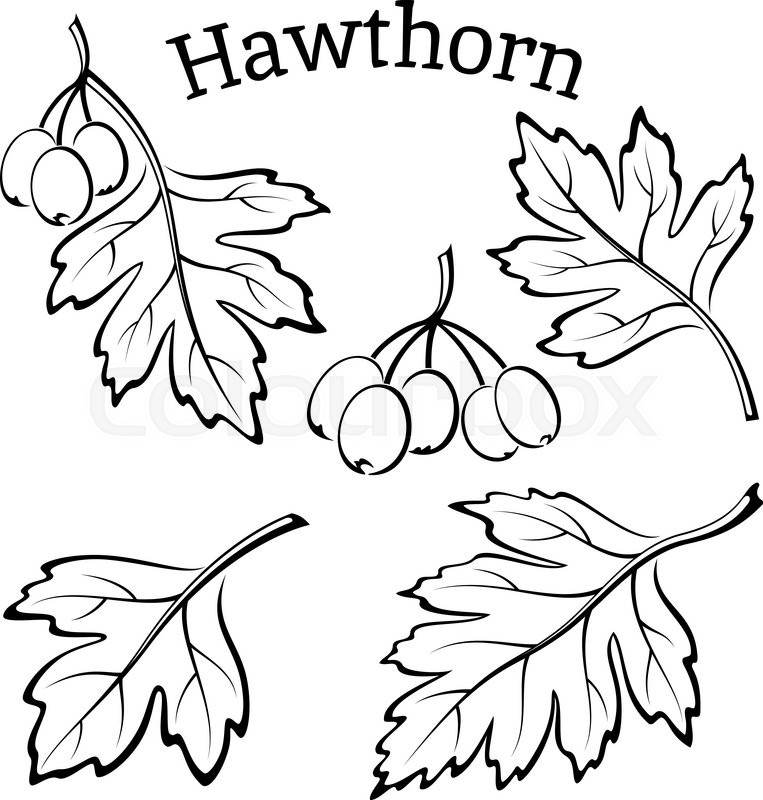This black and white image resembles a detailed coloring page. At the top center, the word "Hawthorne" is prominently displayed in an arched, serif font, with only the "H" capitalized. Below this text, several sketched leaves are arranged in different orientations on a solid white background. In the upper left corner, a large leaf detailed with visible grooves has three outlined, oval-shaped acorns hanging from its tip. The upper right corner features another large, detailed leaf with no acorns attached. In the center of the image, five acorns are clustered together, unattached to any leaf. The lower part of the image contains two more sketched leaves: the lower left corner has a downward-facing leaf, while the lower right corner presents a slightly larger leaf, also facing downward. A barely visible watermark reading "colourbox" in light gray is centered in the background, suggesting the image could be used for coloring.